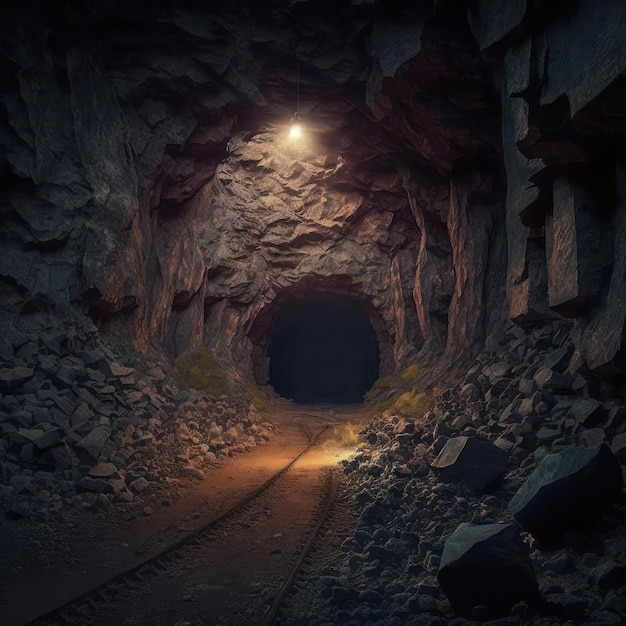This image, presenting as either a highly realistic photograph or a meticulously crafted digital painting, captures an underground tunnel that exudes a sense of mystery and antiquity. The scene is dominated by a round, railway-like tunnel, seemingly too small for a full-size train, suggesting it is part of a mining system. The tunnel extends into pitch-black darkness, concealing what lies within.

The tunnel's entrance is framed by rough, jagged stones and blocks piled haphazardly on either side, with the surrounding rock displaying a blend of brown, reddish, and gray hues. The ground at the entrance is composed of orange-hued soil, interspersed with small, narrow tracks that hint at their use by mine carts. 

Adding to the eerie ambiance, a single light hangs from the cave's ceiling at the very top of the tunnel, casting a yellow-orange artificial glow that barely penetrates the deep blackness beyond. This solitary light only enhances the foreboding atmosphere of this seemingly endless, dark tunnel.